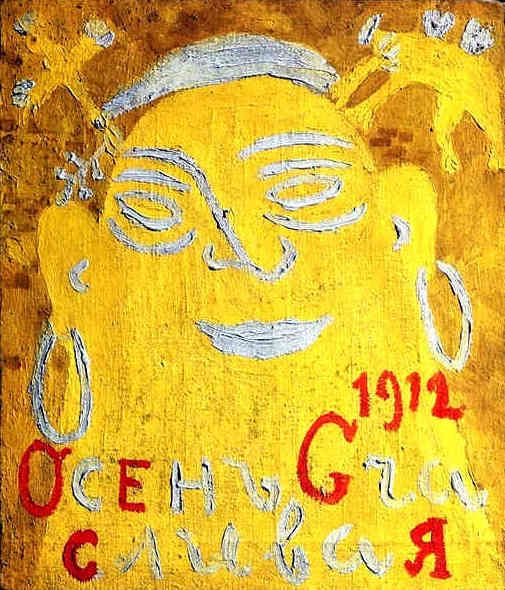The image is a playful and somewhat abstract painting, featuring what appears to be a stylized, rough depiction of a human-like figure, possibly inspired by an African tribal statue or reminiscent of a thumb. The central figure is yellow, blending in with a splotchy orange and brown background that gives the impression of yellow flames or a goldish hue. The figure has a white streak at the top of its head resembling hair, with simplistic facial features: white ovals for eyes with two slashes above and below, a simple hook-shaped nose, and white lips that form a slight smile. Adding to its distinctive look are white hoop earrings. At the top of the figure's head, one can see two protruding forms—a cross on the left and an abstract shape on the right; possibly horns.

Details in the upper corners add further intrigue: the upper left features a small yellow bird flying upwards, while the upper right corner includes a shape resembling a four-legged animal, which could be interpreted as a bull or dog. Beneath the figure are the numerals "1912" in red, perhaps indicating the year of creation, alongside other alternating white and red letters that are partially legible, spelling out fragments like "OCEH G" and "CALLUA" with a reversed 'R'. These scattered letters add a cryptic element to the artwork. Overall, the depiction is both humorous and childlike, yet steeped in abstract symbolism.